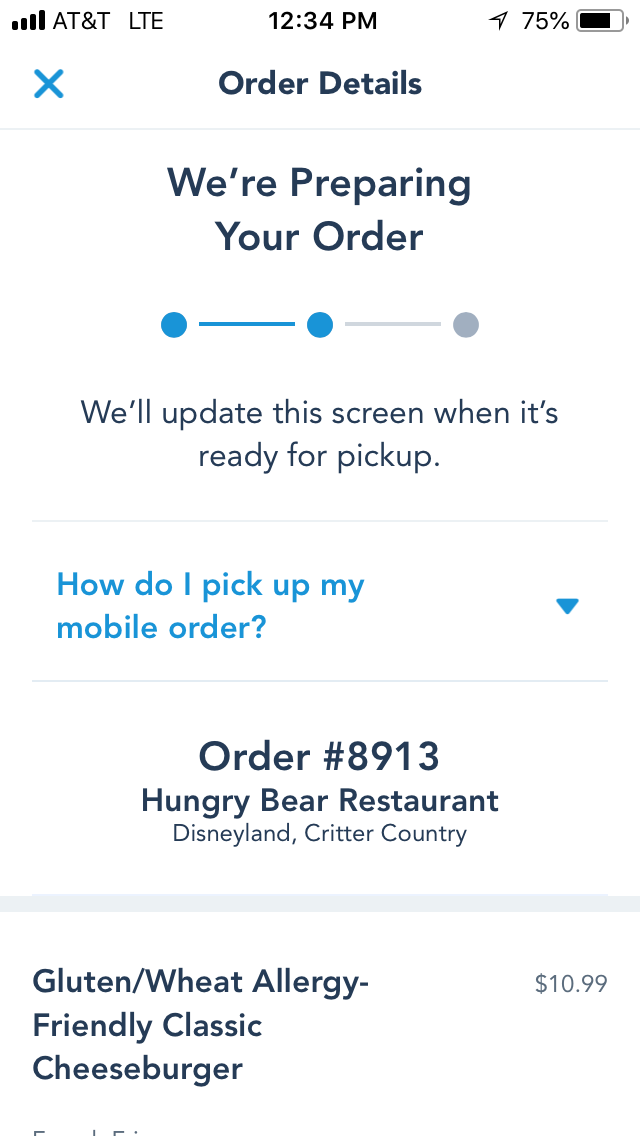This is an image showcasing a screenshot taken from a smartphone. The status bar indicates the device is connected to AT&T LTE, not Wi-Fi, with the time displayed as 12:34 PM and the battery at 75%. The screen shows order details, with a notable 'X' mark at the top. 

The order is currently being prepared, as indicated by a progress bar consisting of a circle connected by a line to another circle, both of which are solidly filled in. The screen informs that updates will be provided when the order is ready for pickup. 

Below this information is guidance on how to pick up a mobile order. Scrolling further reveals the order details: Order number 8913, made at Hungry Bear Restaurant located in Disneyland's Critter Country. The order is for a gluten and wheat allergy-friendly classic burger (cheeseburger), priced at $10.99.